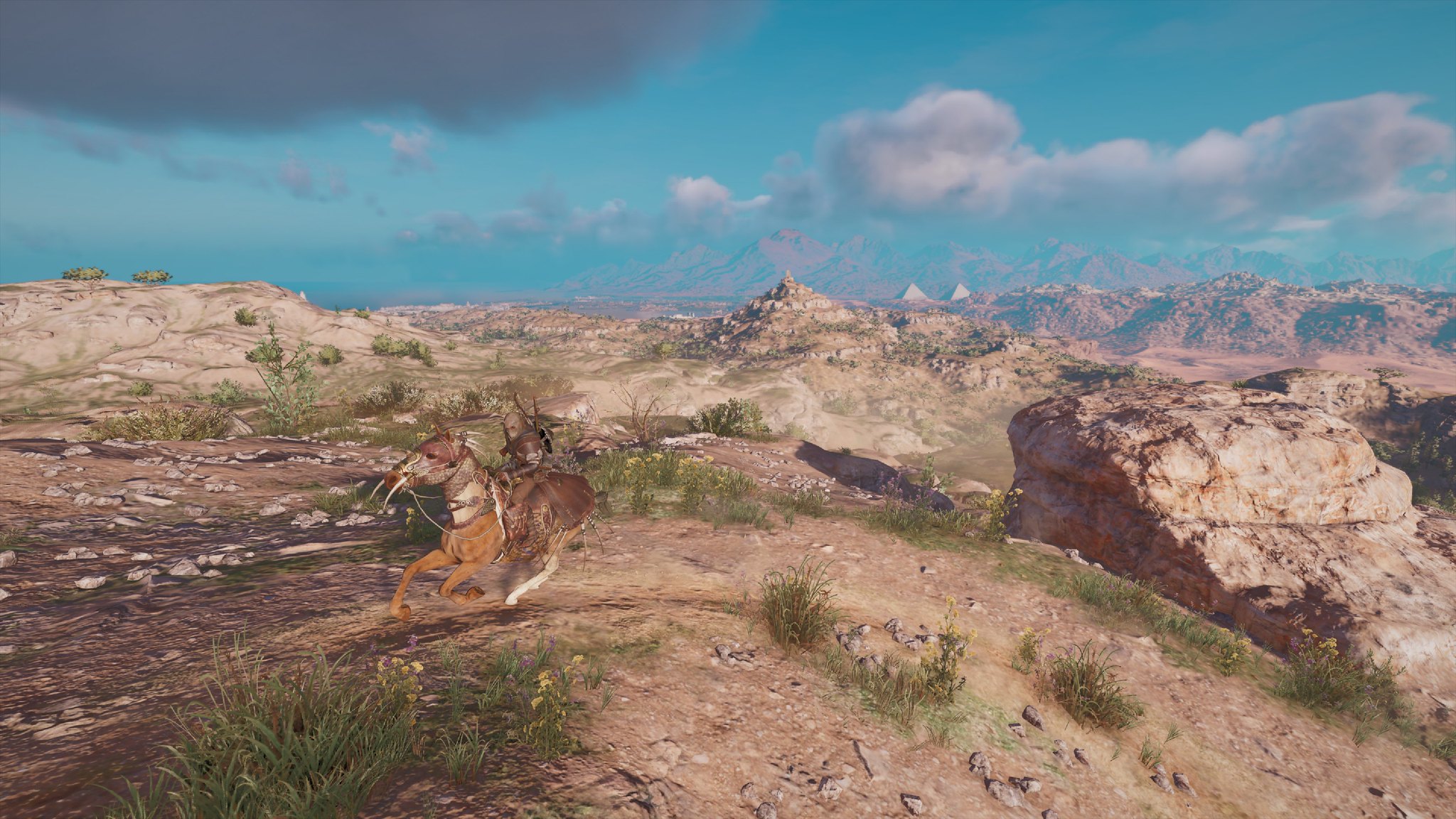In this captivating wide-angle photograph, a surreal and intriguing creature can be seen dashing towards the right side of the frame within a picturesque, rocky mountainous region. This enigmatic animal, a curious blend resembling a fusion of a dog, a horse, and a saber-tooth tiger, features a body fraught with contradictions. It has short stature akin to a dog and sports brown legs with a distinctive white marking on one of its hind legs. Its face, reminiscent of a horse, is adorned with two prominent tusks protruding from either side of its mouth, creating an almost mythical appearance.

There's an ambiguity about the creature's back – it either appears to be wearing a saddle or could be chewing on something, possibly another animal. The image's wide-angle lens might be attributing to this creature's distorted and fantastical appearance.

In the background, a stunning mountainous range stretches across the horizon towards the right, adding depth and majesty to the scene. The foreground is dominated by a significant rock formation located in the bottom right corner, adding texture and dimension to the landscape. The ground beneath this creature's rapid movement is a rugged mix of dirt, rocks, and sparse patches of grass. Overhead, a bright blue sky with scattered clouds completes this striking natural tableau.